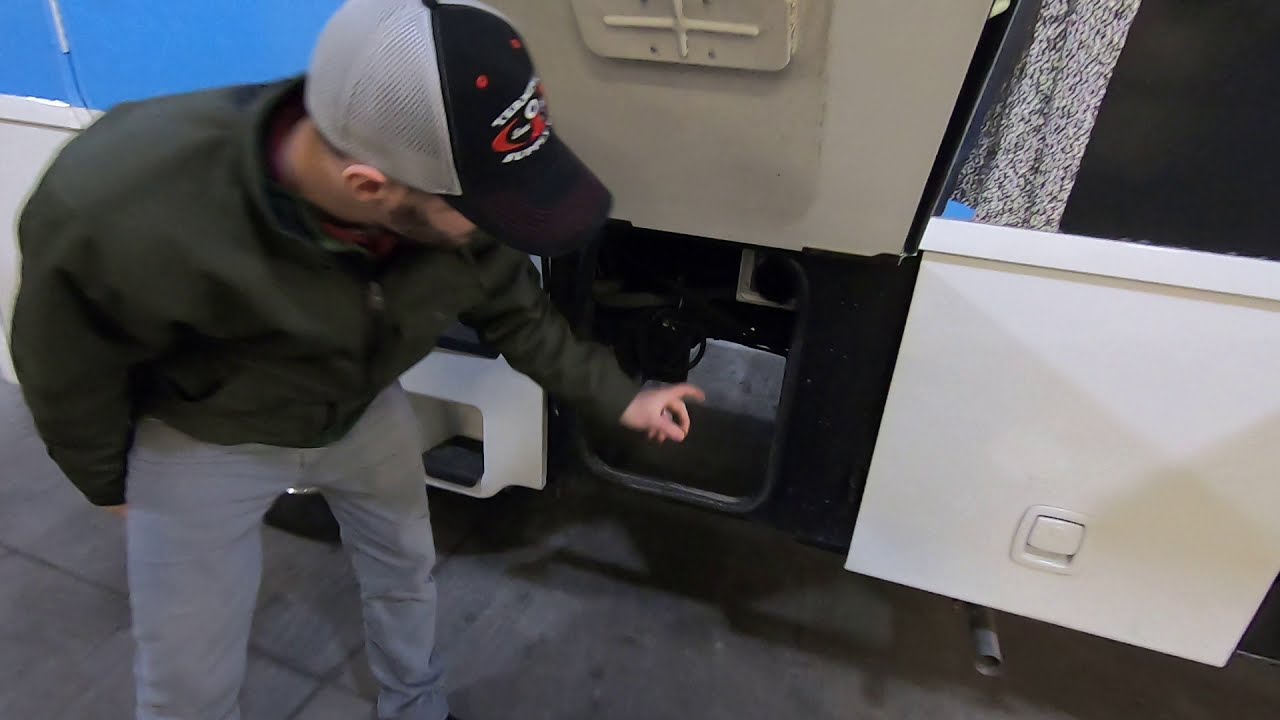The photograph depicts a white male with a black beard and wearing a black brimmed baseball cap featuring white netting at the back and a white and red logo on the front. He is attired in a dark zip-up coat, which appears brownish gray in some lights, and light blue, somewhat faded jeans. He is crouched down and focused on an open compartment along the side of what appears to be a semi tractor-trailer truck, although it could also be an RV or motorhome as suggested. The truck or vehicle in question is painted blue and white. The man is supporting the hatch, possibly with his shoulder, while pointing at an inner component of the compartment, which might be related to an electrical or gas system, or perhaps checking the water level or generator. The image is slightly blurry, and the man’s face is concealed as he intently examines the area he’s interacting with.